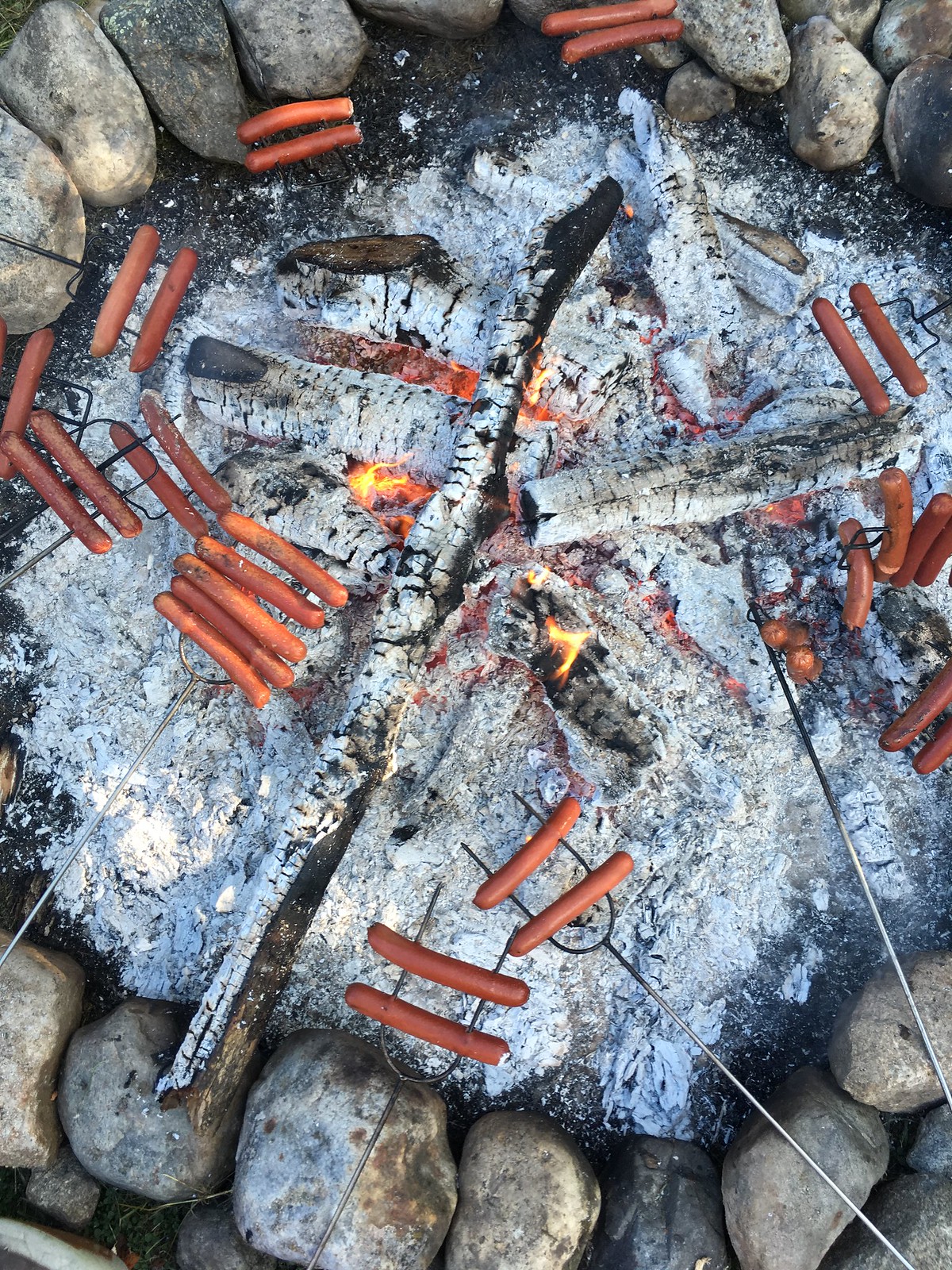This image is a bird's-eye view of an outdoor fire pit surrounded by large gray rocks, forming a rugged circle which contains partially burnt logs covered in a thick layer of white ash. The central focus is on the glowing embers and small flickers of flames within the pit. Around the fire, multiple skewers (at least ten) with two to six hot dogs each are extended from all directions, held by unseen people presumably cooking their meal. The skewers are equipped with two tines each, some positioned closer to the fire, indicating that the cooking process has just begun; none of the hot dogs appear cooked yet. This scene likely depicts a group gathering, possibly during a camping trip, enjoying the communal activity of roasting hot dogs over a long-burning, well-maintained fire.